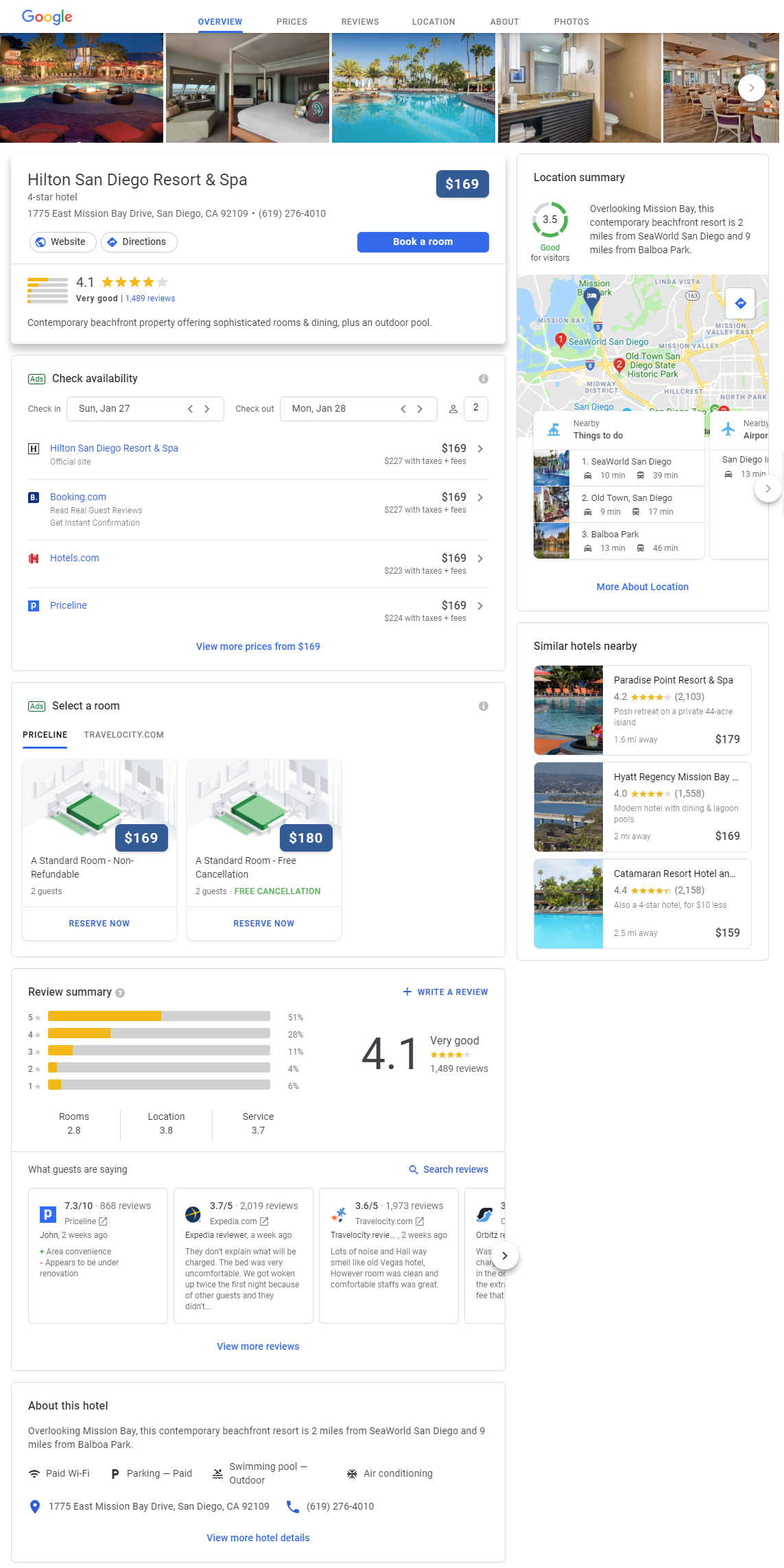This image is a screenshot of a hotel advertisement, likely captured on a mobile device due to its vertical orientation. The header features the Google icon, indicating this information is sourced from Google, with various tabs visible such as Overview, Prices, Reviews, Location, About, and Photos, with the Overview tab currently selected.

The main content area displays five images showcasing different aspects of the hotel: a swimming pool, a bedroom, a bathroom, and a breakfast area, providing a glimpse into the hotel's amenities and environment. Directly below these images, a box highlights the "Hilton San Diego Resort and Spa" with room prices starting at $169. It also mentions that the hotel has received a rating of 4.1 stars from 1,489 reviews, suggesting a generally positive reception from guests.

A "Check Availability" button is prominently placed to facilitate booking, alongside an option to "Select a Room," which offers a detailed view of room schematics, pricing, and photographs, enhancing the booking experience by allowing potential guests to visualize their stay.

In the upper right corner, a location summary is provided with a map, powered by Google Maps, pinpointing the hotel's location. Nearby attractions, such as SeaWorld San Diego, are also indicated, making it easier for potential guests to plan their visit. Below this map, there is a section listing similar hotels nearby, offering additional choices for accommodation.